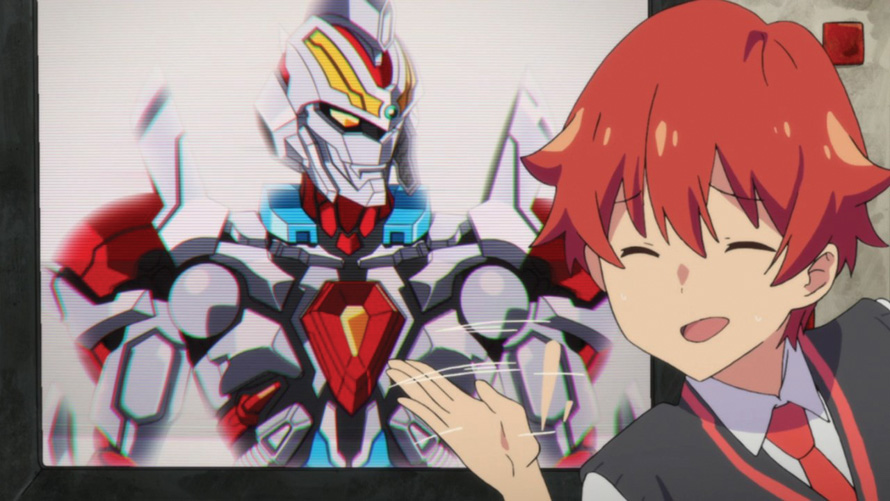The image depicts a detailed cartoon scene set against a predominantly white background. On the left side of the image, a Transformer-like robot is shown in its combat form. This imposing robot is primarily gray with intricate details and mechanical texture, accentuated by bolts and design lines. The robot's head is gray, with striking yellow eyes that feature red pupils. The sides of its head are yellow, while the central portion, including the neck area, is red with subtle blue highlights.

In front of this mechanical giant stands a young boy with brown hair. He appears to be waving, creating a sense of interaction with the robot. The boy is dressed in a formal outfit: a white shirt paired with a red tie, and a dark gray or black vest. The juxtaposition of the boy's animated gesture against the robot's stoic stance adds an engaging dynamic to the scene.